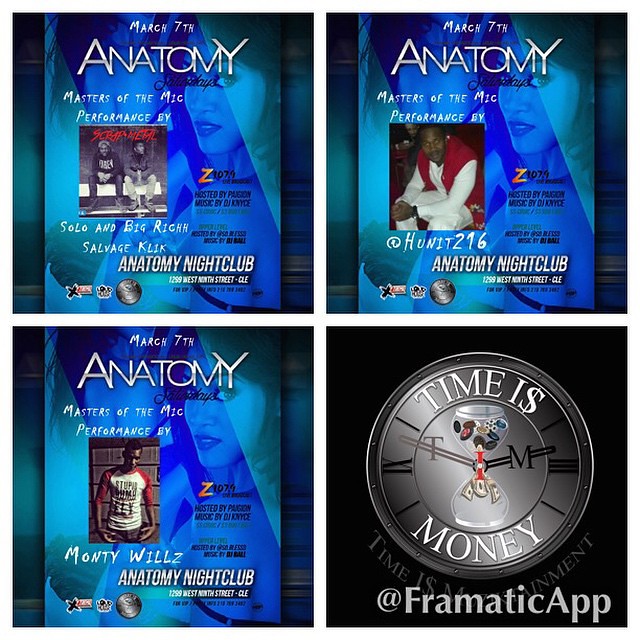This is a vertical rectangular image collage composed of four square images arranged in a 2x2 grid. The upper row features two promotional flyers for Anatomy Nightclub, while the bottom row includes a third Anatomy Nightclub flyer on the left and a distinct promotional image on the right.

The top left flyer announces "Masters of the MIC" event on March 7th at Anatomy Nightclub, showcasing a performance by two men seated on a white bench, with their names listed as "Solo" and "Big Rich." A blue background features a faint image of a woman, consistent across all three nightclub flyers. The top right flyer mimics the left but with a different performer, "Hunit 216," against the same blue-themed backdrop.

The bottom left flyer follows the same design but highlights a performer named "Monty Wills." All three nightclub flyers share a similar aesthetic with a dark blue background and a superimposed image of a woman, enhancing the nightclub's branding consistency.

In contrast, the bottom right image stands out with a black background and a clock face comprising Roman numerals. An hourglass icon, possibly symbolizing urgency or limited time, is centered on the clock. The upper arc of the clock reads "Time is," and the lower arc states "Money." Below, it directs viewers to "@framaticapp," presumably where the watch can be obtained.